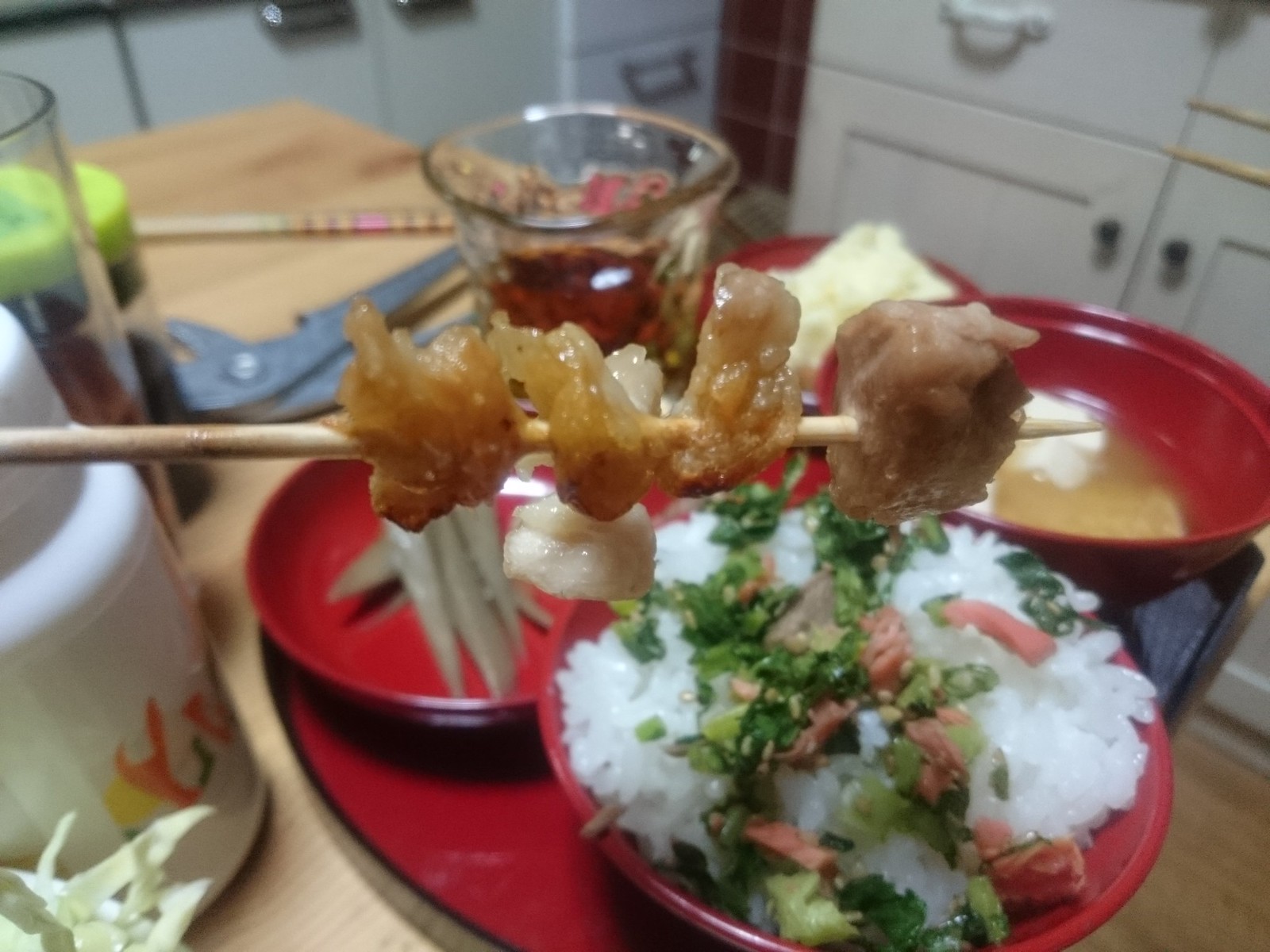On a rustic butcher block table sits a vibrant spread served in three red bowls on a matching red circular tray. The centerpiece is a tantalizing kebab, skewered with four succulent shrimp, held above the bowls. Just below the kebab, one bowl contains a bed of white rice adorned with salmon-colored pieces of meat and sprinkled greens. To its right is a bowl of tan-colored broth, and to the left, a bowl with thin, gray, delicate strips of food. A glass container with a medium brown sauce sits behind the kebab, accompanied by a jar with a yellow lid in the upper left corner. The table also features a glass of wine, adding to the inviting ambiance. In the background, white cabinetry frames the upper left and right, enhancing the cozy, homely setting of this appetizing meal.